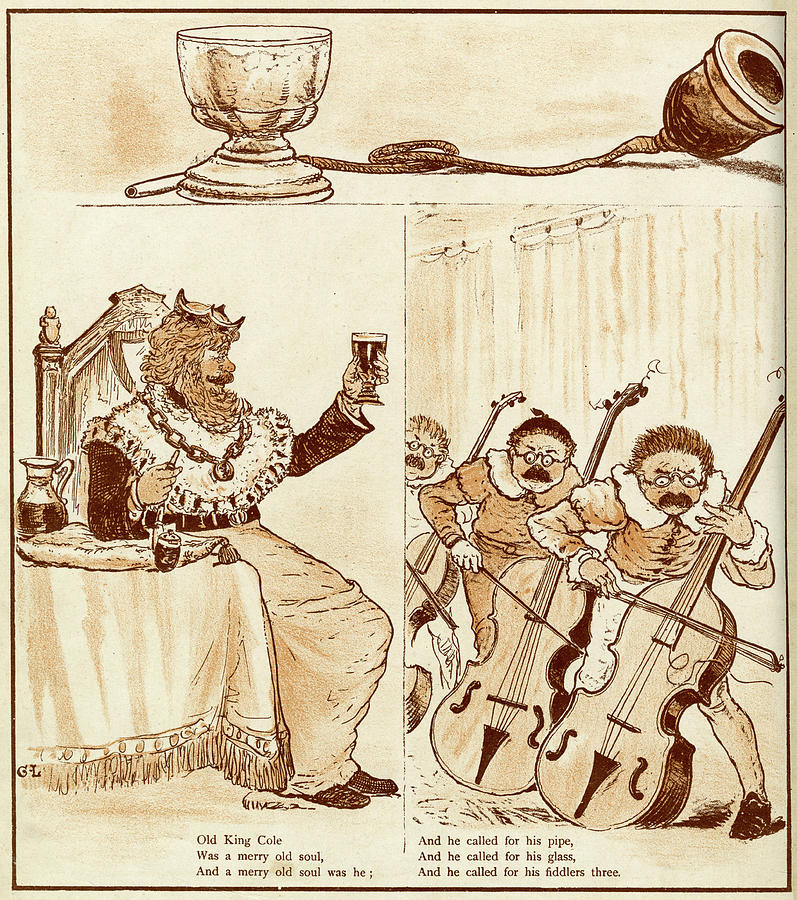The animated sketch, set against a pinkish background, is divided into three distinct parts. At the top, there's a small gray, white, and black comic book-style illustration featuring a metallic bowl with a string and an adjacent pipe. Below this, occupying the left-central portion of the image, is a detailed depiction of a jovial king, labeled as Old King Cole. He is seated on an ornate chair, adorned with a large gold chain, a crown, a long beard, and a fur mantle. In his left hand, he holds a raised goblet, while his right arm rests on a table covered with a pink tablecloth, which also holds a pitcher of liquid. To his right, taking up the remaining right-central part of the picture, are three musicians, who, despite varying descriptions, appear consistent in having identical mustaches, short haircuts, and peculiar glasses. They are energetically playing their instruments, which resemble either fiddles or cellos. Below this central scene, the text reads, "Old King Cole was a merry old soul, and a merry old soul was he; he called for his pipe, and he called for his glass, and he called for his fiddlers three."